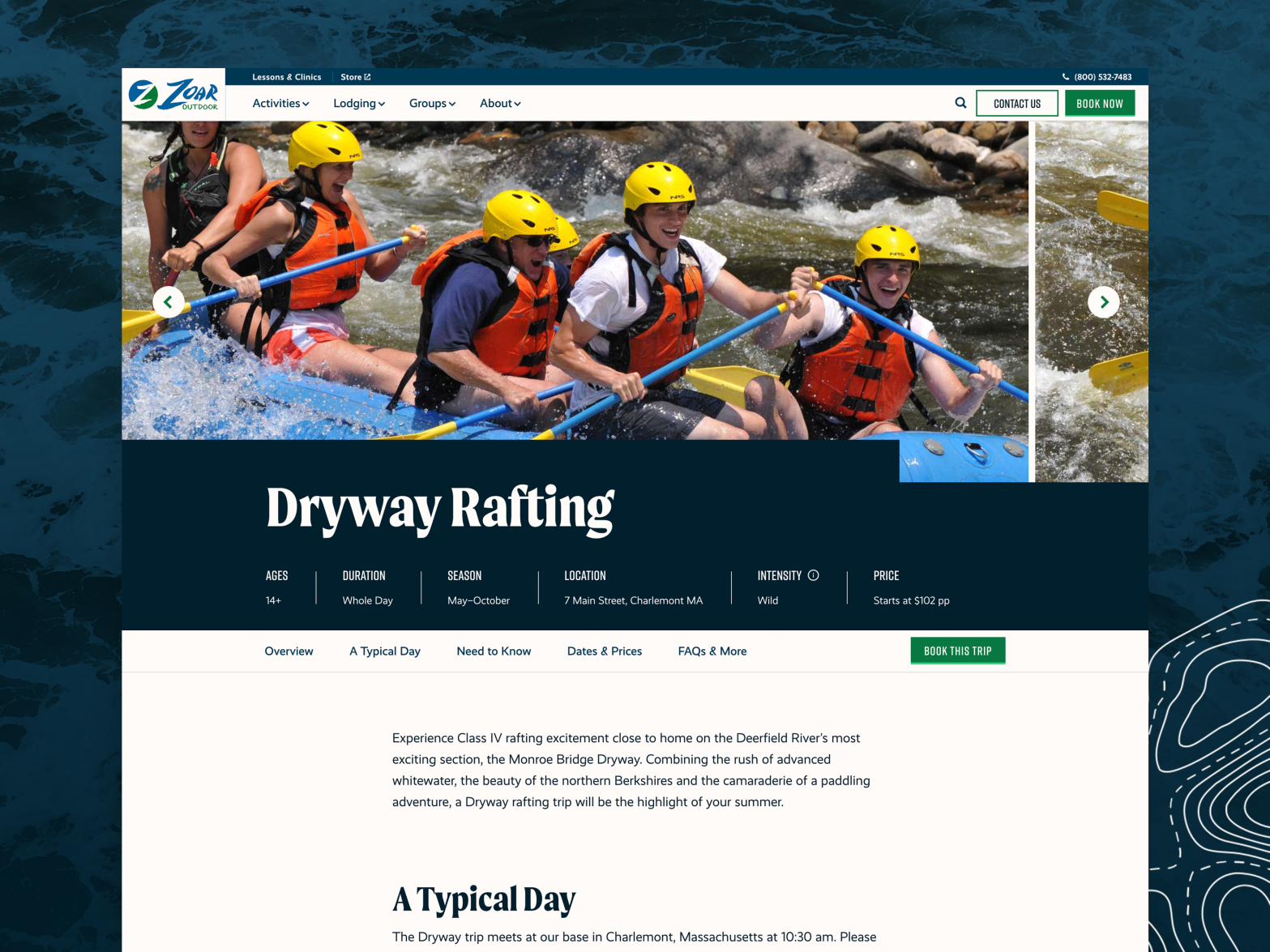The image captures an exhilarating scene of a family white-water rafting on the Deerfield River, characterized by its intense class 4 rapids. Prominently highlighted in the upper section of the image is a blue banner featuring the logo "Xeor Tours," with navigation options for "Activities," "Lodging," "Groups," and "About" clearly presented in a small white box.

Beneath this banner, the family is visibly engaged in the rafting adventure, each member equipped with yellow helmets and life jackets for safety. The joy and thrill of the experience are palpable as they navigate the wild waters.

Further details are provided in a detailed caption below the picture, which describes the activity as "Driveway Rafting," suitable for individuals aged 14 and up. The full-day event runs from May through October, starting at 7 Main Street, Claremont, MA, with prices beginning at $202 per person. The activity is noted for its high-intensity excitement and promises an unforgettable experience.

An additional green box invites viewers to "Book this Trip," emphasizing the unique opportunity to enjoy an advanced white-water rafting adventure combined with the scenic beauty of the northern Berkshires. The text notes that the typical day starts at the tour base in Claremont, MA, at 10:30 AM, but cuts off mid-sentence.

Overall, this image and its accompanying details vividly promote an adventurous and scenic white-water rafting experience offered by Xeor Tours.